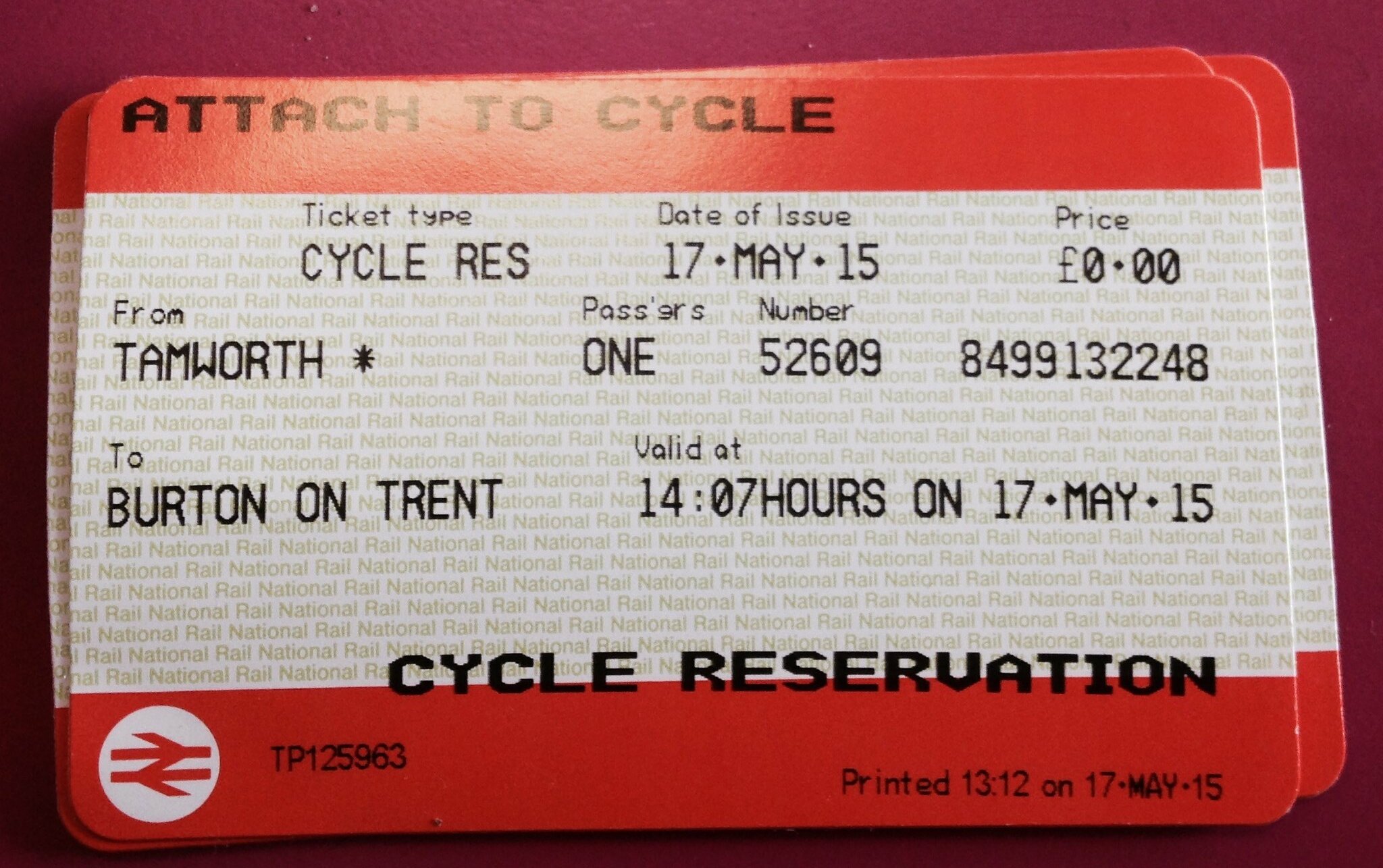This image is a rectangular photograph capturing a stack of cycle reservation cards, arranged on a reddish-purple table. The top card, identical to the ones underneath, is prominently displayed and features red stripes across the top and bottom, with the main body of the card being white. In black text, it begins with "attached to cycle" at the top left. Below, the bulk of the detailed information is printed, including the ticket type labeled as "cycle reservation," the date of issue as "17 May 15," and a note that it is valid for one passenger traveling from Tamworth to Burton-on-Trent. The price is listed at zero pounds. A unique number sequence "five two six zero nine" and "eight four nine nine one three two two four eight two" appears on the card. The card is valid at 14:07 hours on the same date. The background also features a repetitive, faded "National Rail" print. At the bottom right, in larger black letters, it reiterates "cycle reservation," and provides a printed time of "13:12 on 17 May 15," alongside additional coding and the National Rail logo on the left.